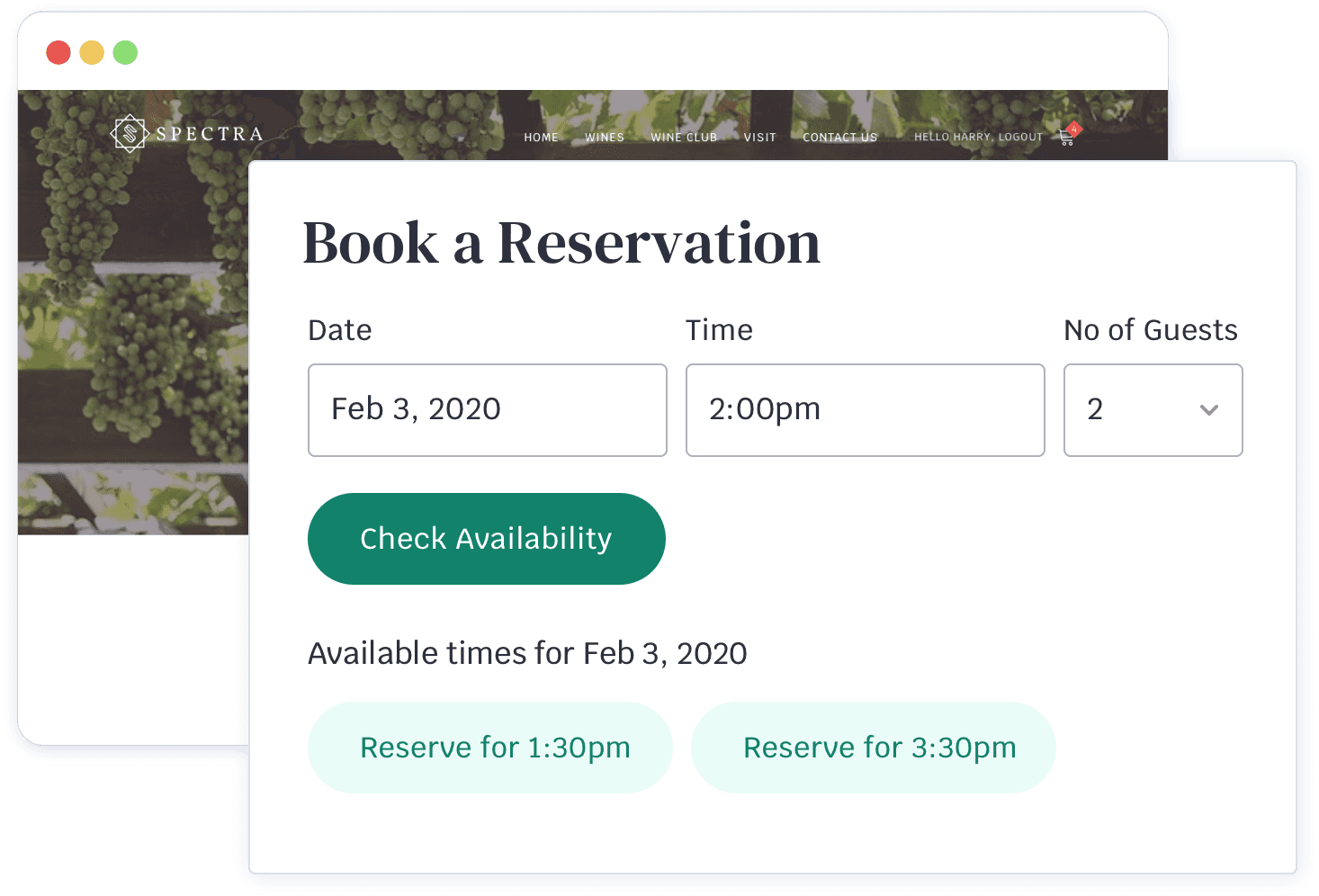The image displays a reservation booking popup on the Spectra website, partially obscuring the main content. The popup has a rectangle shaped horizontally longer than vertically, with a white background. At the top in large font, it says "Book a Reservation." Below that, there are three horizontal fields for selecting the date, time, and number of guests. The "Date" field is pre-filled with "February 3rd, 2020", the "Time" field with "2 p.m.", and the "Number of Guests" is set to "2" with a dropdown menu for adjusting the count.

Adjacent to the date field on the left side, there is a dark green button labeled "Check Availability" in white text. Below these fields, the popup displays the availability status for the selected date with another heading that reads "Available times for February 3rd, 2020" in black text. Two light green buttons for available reservation times follow underneath: one button saying "Reserve for 1:30 p.m." in dark green text and the next one stating "Reserve for 3:30 p.m." in the same style.

The background of this popup is entirely white and it obscures most of the Spectra website except for the navigation bar at the top. The navigation bar, overlaid on a photograph of vineyards with hanging grapes, has a white background and includes the following menu options: "Home," "Wines," "Wine Club," "Visit," "Contact Us." There are also user-specific elements such as "Hello Harry," "Log Out," and a cart icon with a red box on it.